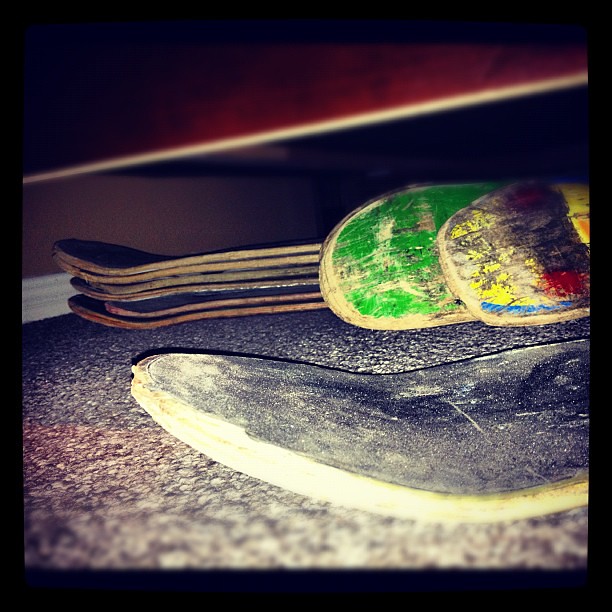This real-life photograph captures a close-to-the-ground view of a dimly lit, carpeted room with a dark brown wall in the background. Centered in the scene are several skateboard decks in varying conditions and orientations. In the background, along the baseboard of the wall, there is a stack of skateboard decks piled at least six high, though details are hard to make out beyond the top one due to the shadowing and blurriness. Two well-worn skateboards lay on their sides in front of this pile; one deck is primarily green, while the other features a yellow, red, and blue pattern. The foreground is dominated by the end of another skateboard deck, appearing black, dusty, and particularly worn, exposing the underlying wood. The photograph is framed with a black border, and some of the shadows and reflections suggest the use of a flash close to the camera.